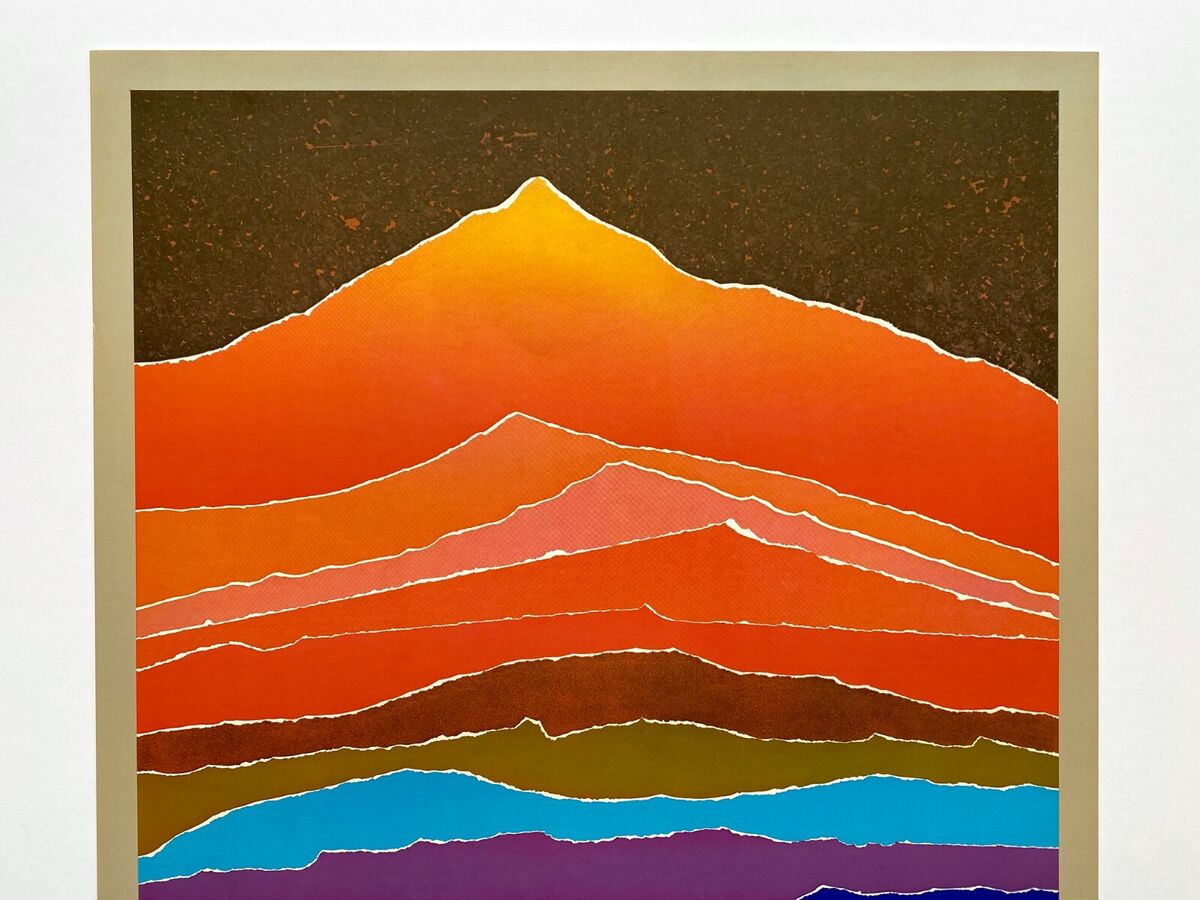The image is a large square artwork set against a light gray background. At the center, there's a picture frame with a thick gold border on all sides except the bottom. The artwork inside appears to be a multi-layered piece, possibly utilizing layers of paper. The top section depicts a sky rendered in dark brown with speckles of orange. Below this, a series of painted mountain peaks, outlined in thin white lines, cascade downward. The foremost peak, which is the largest, rises sharply before tapering downwards. The peaks are shaded in varying hues of orange, with the topmost having a lighter orange tip. As the image progresses downward, the mountain shapes transform into v-shaped strips of orange, decreasing in thickness. The color transitions fluidly from brown at the top to green, blue, and finally purple at the bottom. The intricate detailing and layered effect give the impression of the diverse and vibrant topography of what might be the Piton Mountains.